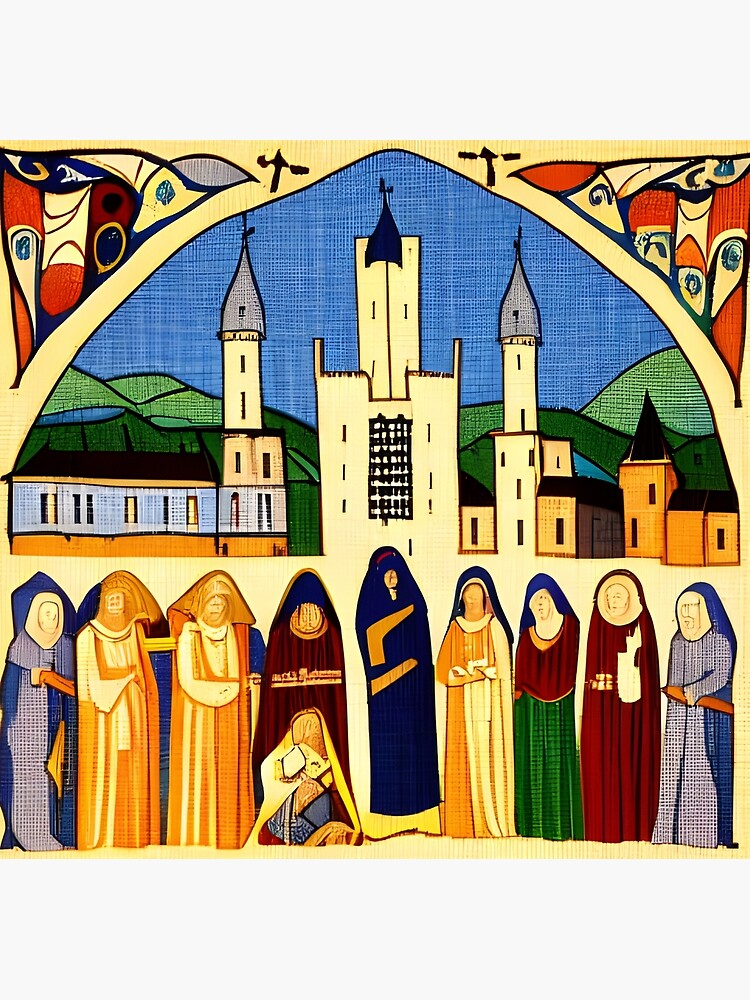This artwork, potentially an oil painting or embroidered tapestry, vividly depicts a religious scene with intricate details. The central focus is a white or yellow church with a tall steeple topped by a cross, framed by two towering, spired structures on each side. The background reveals a blue sky and rolling green hills. The top of the image is adorned with geometric, abstract patterns in red, orange, purple, and blue, forming an arch that encapsulates the scene.

Beneath the arch, the artwork features a group of nine religious figures, possibly nuns or holy women from ancient times, arranged in prayerful postures. They are dressed in a vibrant array of colors, including red, yellow, orange, blue, green, and burgundy. Among them, one woman kneels, draped in a yellow veil and blue dress, cradling an infant child as the others look down at her reverently.

The left and right sections of the artwork include additional village buildings and significant religious iconography, such as embroidered crosses and abstract shapes, enhancing the sacred atmosphere. The absence of any textual elements allows the visual narrative to convey the solemn and devout essence of the scene.